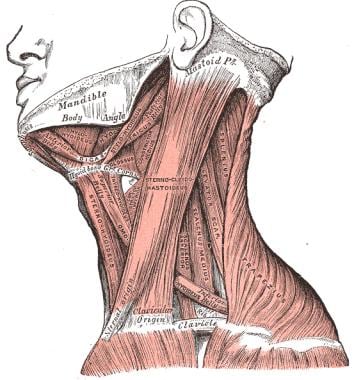The image presents a detailed anatomical sketch of the human neck, set against a completely white backdrop. It spans from just below the nose to the clavicle, depicting a cross-sectional view of the muscles, tendons, and bones in that area. The head is partially visible, with features such as the bottom of the nose, ear, mouth, and the contour of the face, all illustrated in black and white. The muscles are predominantly colored in red, with intricate striations, while the ligaments and tendons appear in white. The upper jaw and mandible are highlighted, with labels such as "mandible" and "mastoid" placed in strategic locations to denote key anatomical structures. The mandible is prominently labeled in the upper left corner of the image. Additional labels and writing are present on various muscles, although not all text is legible due to the resolution. Notable muscles like the trapezius and sternocleidomastoid are clearly depicted, including their connections to the clavicle and mastoid insertion at the base of the skull. The overall image, reminiscent of a medical textbook diagram, offers a comprehensive view of the neck’s musculoskeletal architecture.